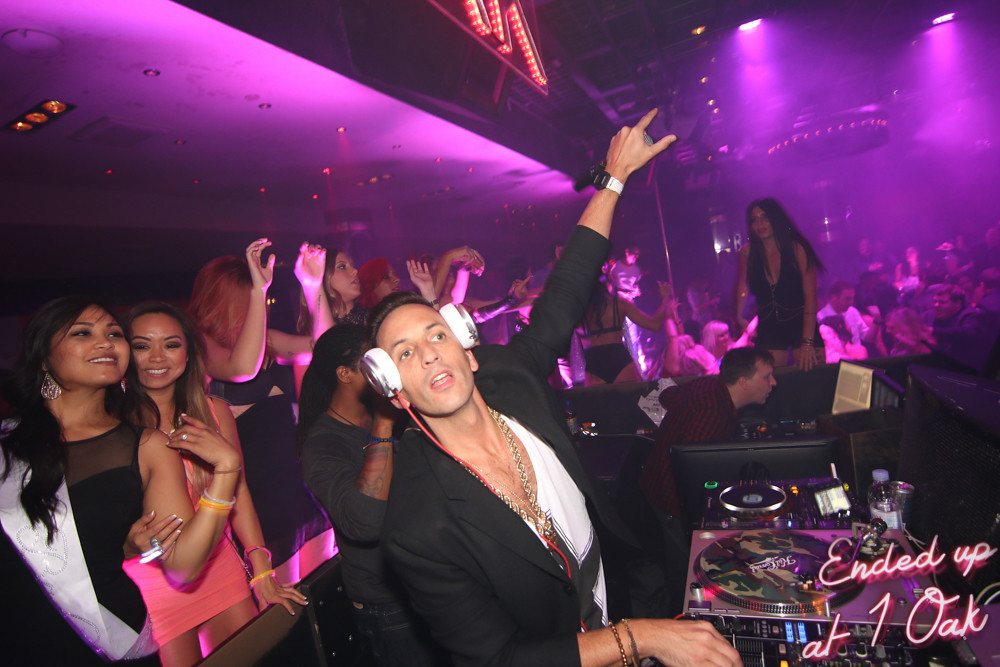In the vibrant, pulsating atmosphere of a nightclub, a DJ stands at the forefront, highlighted with his left hand raised energetically as he spins tracks on his equipment. The DJ, adorned with a gold chain, a dress jacket over a white t-shirt, and large white headphones, exudes a commanding presence. Behind him, a sound engineer, clad in a black and red flannel shirt, intensely focuses on his computer. To the left of the DJ, the dance floor bathed in pink and purple lighting comes alive with numerous women dancing, smiling, and posing for the camera. The scene is a cacophony of motion and color, underlined by the neon, cursive text in the bottom right corner, reading "Ended up at One Oak," encapsulating the lively night.